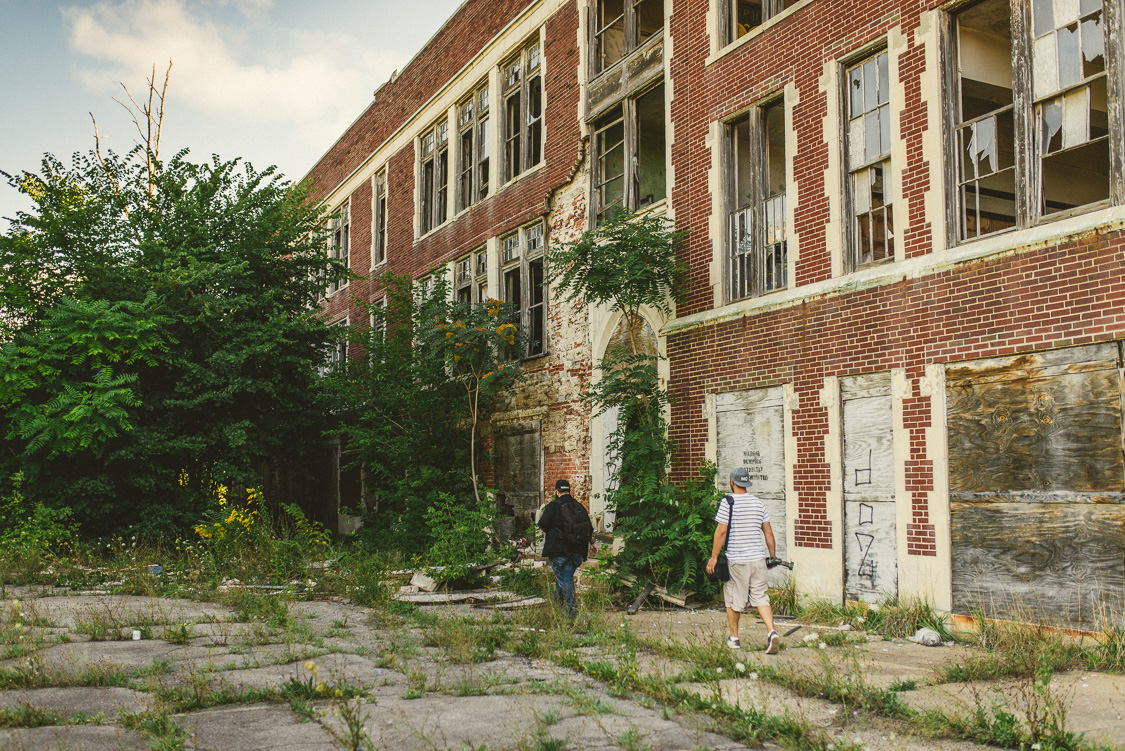The image captures a deteriorated, abandoned building, likely an old factory or possibly a school, made primarily of red brick with white trim. This three-story structure is riddled with broken windows, and many doorways and windows are boarded up with particle board covered in graffiti. Parts of the wall are missing, indicating substantial neglect. The surrounding area, which once might have been a paved parking lot or pathway, is now cracked and overrun with grass and weeds. A large tree or bush is visible on the left-hand side, and vines creep up the building's walls.

Two men, presumably photographers, are seen from behind, walking away from the camera and scouting the area. The first person wears a black jacket, blue jeans, a black hat, and a black backpack. The second person, slightly to the right, dons a gray backwards hat, a white and gray striped shirt, tan cargo pants, and skate shoes. He carries a camera in his right hand and has a black camera bag draped over his left shoulder. The sky above is cloudy with patches of blue, hinting at a somewhat overcast day.